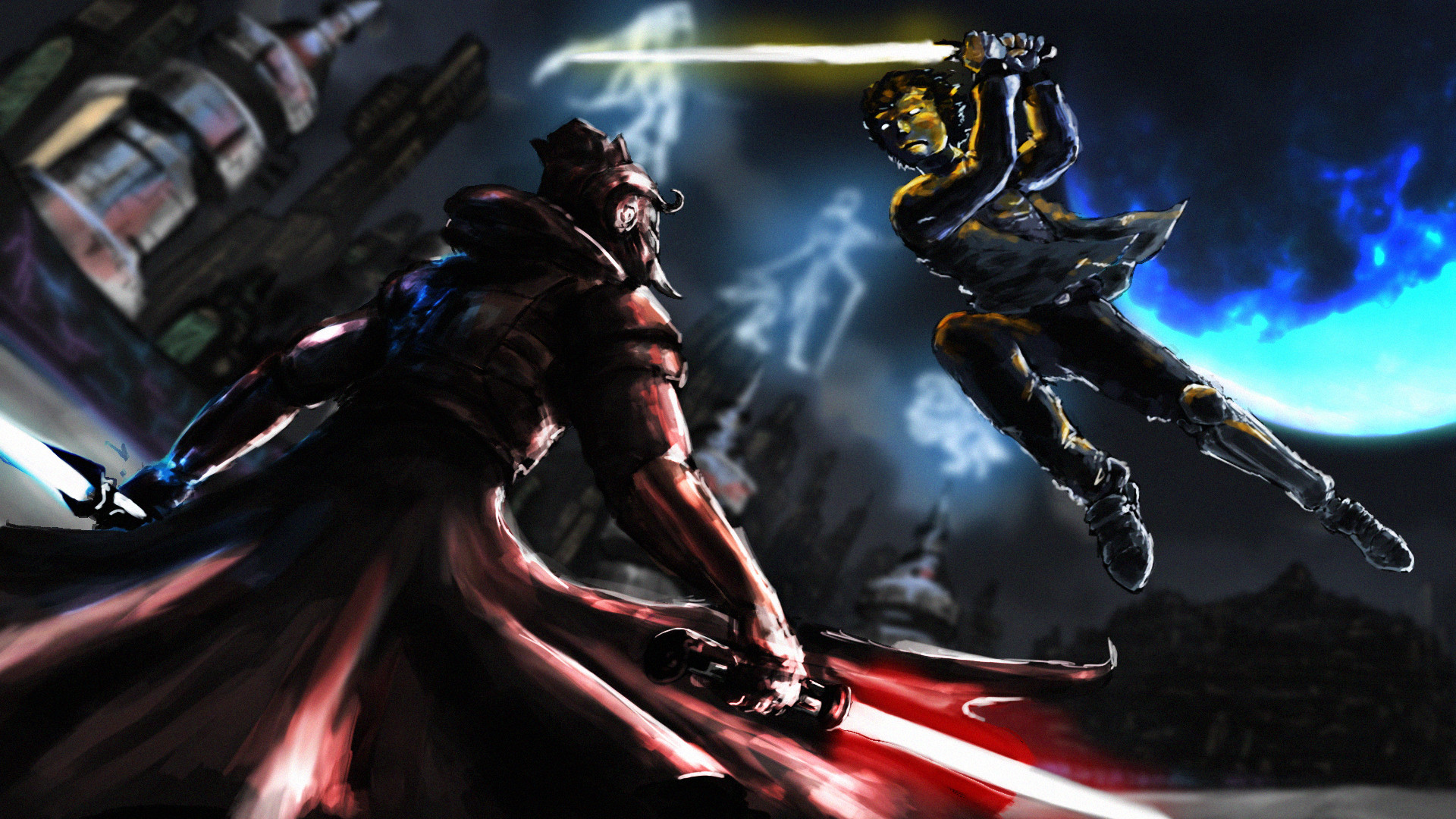The image is a detailed sci-fi painting capturing an intense combat scene between a hero and a villain. The hero, a leaping figure with a blurred face and indistinct facial features, brandishes a white lightsaber that casts an ethereal yellow glow reflecting off his attire. In contrast, the villain stands grounded and poised, wielding two lightsabers—one red and one bluish. Both characters are set against a backdrop of a tilted, futuristic cityscape. The sky above them is strange, filled with ethereal skywriting-like images that emerge from the spires of three distinct buildings. There is also a wormhole or portal visible behind the airborne hero, adding to the painting's surreal and otherworldly atmosphere. Despite the overall darkness of the scene, the vivid lightsabers illuminate their surroundings, highlighting the dynamic energy of this epic confrontation.